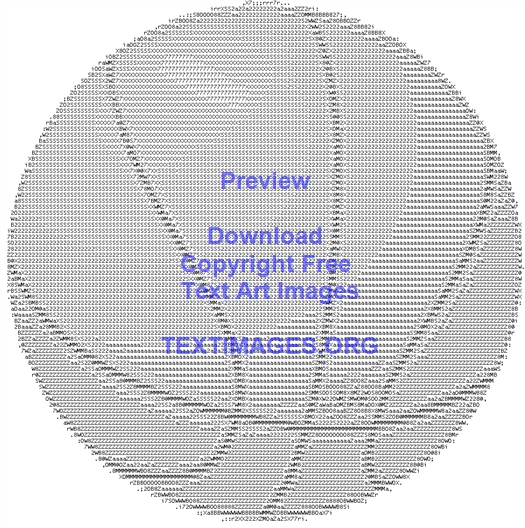This is a square digital artwork featuring a computer-generated graphic of a basketball on a white background. The basketball, composed of various letters and numbers, including B, O, Z, W, and 500, with numerous 2s and Zs, showcases intricate detailing. The black symbols form an image of a basketball, complete with distinctive black lines and artisanal seams made of densely packed characters. The ball appears gray and somewhat degraded in texture, creating a lo-fi effect. At the center of the graphic, light blue text reads "PREVIEW DOWNLOAD COPYRIGHT FREE TEXT ART IMAGES," followed by "TEXTIMAGES.ORG" in all caps. The use of letters and numbers adds a unique, textured appearance to the image.